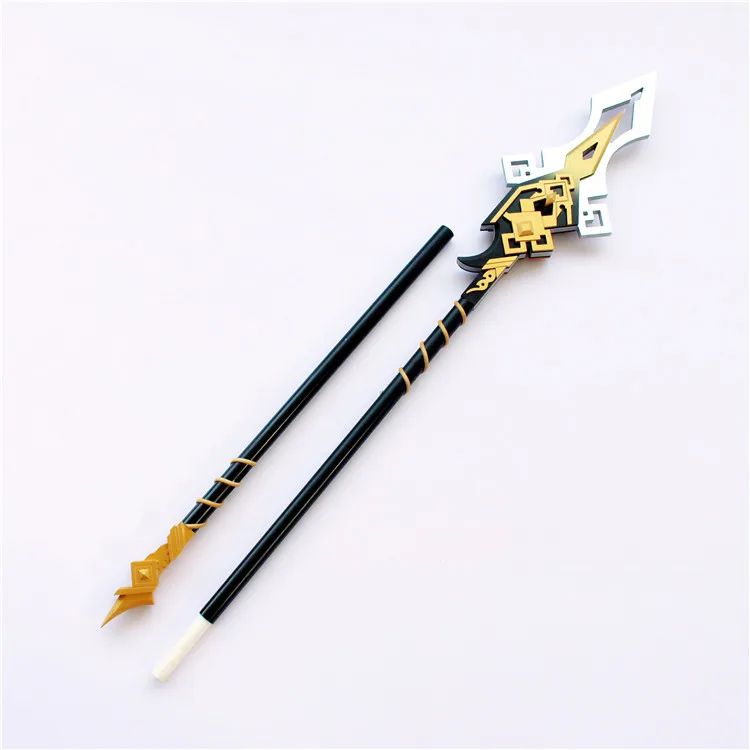The image features two intricately designed black lacquered sticks with gold accents, set against a plain white background, likely photographed in a light box. The first stick is shorter, adorned with a gold design near its extremely pointed tip, reminiscent of a fountain pen. The second stick is longer, also black lacquered with a gold stripe near the tip, and features a more elaborate top section. This ornate top is described as a carved, wood-like, geometric design in gold on a black background, edged with silver, while the bottom end finishes with a white tip. Both sticks bear a prestigious and elegant appearance, combining black, gold, and white in a striking contrast that suggests high craftsmanship, possibly evoking images of marching band paraphernalia or the hands of an ornate clock. The sticks are positioned diagonally from the bottom left to the top right of the image.